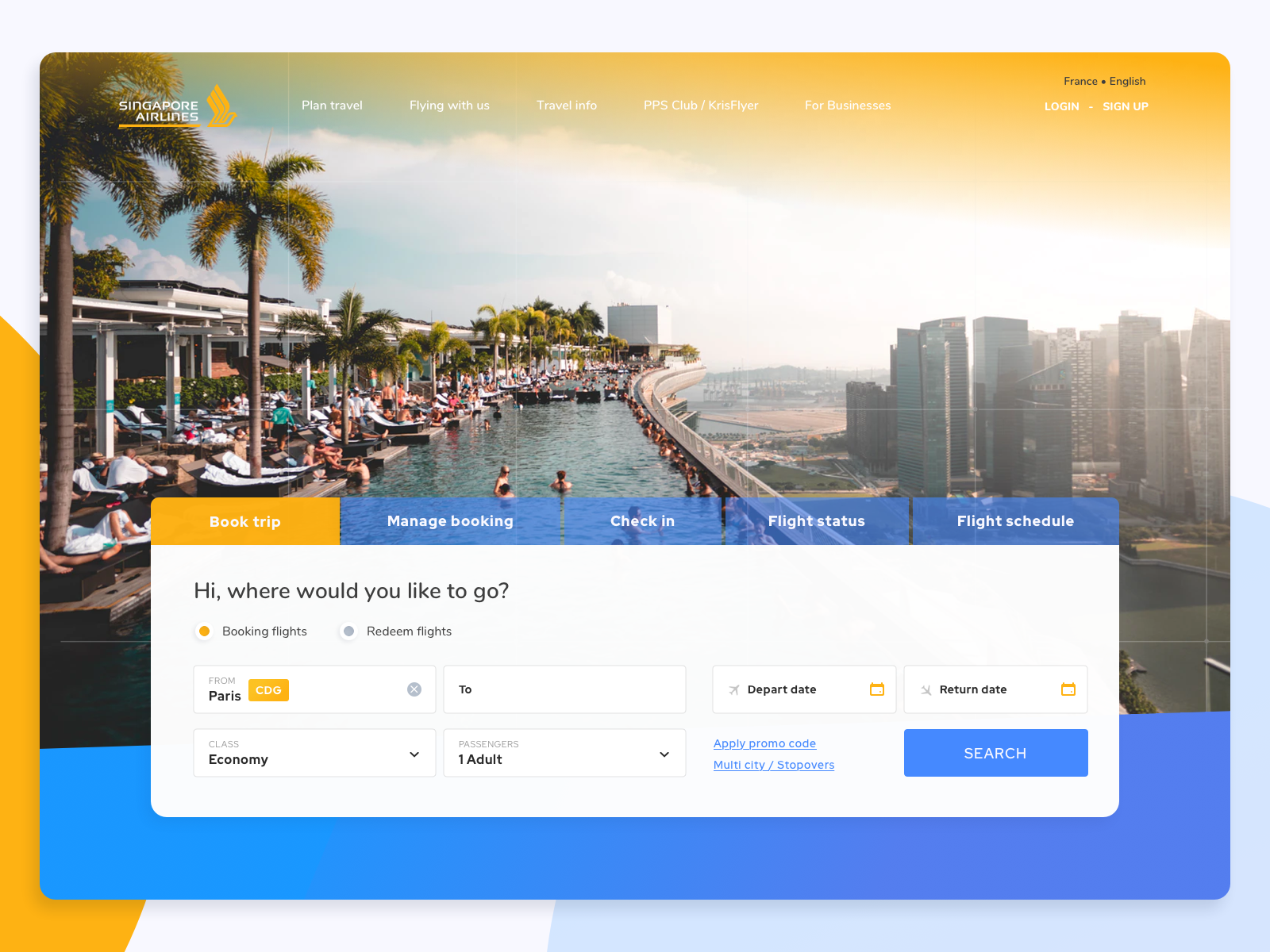**Screenshot of the Singapore Airlines Website**

The screenshot presents a sophisticated and visually appealing website interface for Singapore Airlines. Set in a landscape orientation, the webpage features vibrant colors that make the design elements stand out. Dominating the top portion is the Singapore Airlines logo, displayed in all caps with white text, alongside the well-known logo: a side-view silhouette of a yellow bird in flight.

The navigation bar at the top includes several tabs: "Plan Travel," "Flying with Us," "Travel Info," "PPS Club / KrisFlyer," and "For Businesses." In the top-right corner, users have options to "Log In" or "Sign Up," and there's a language selection toggle between "France" and "English," curiously misrepresented as "France" instead of "French."

The background features a stunning photograph of the renowned Marina Bay Sands hotel, famous for its rooftop infinity pool. Palm trees line the pool area, giving it the appearance of a resort, although it is set atop a skyscraper with the Singapore skyline visible in the distance, creating a breathtaking scene.

Further down the page, the primary functionalities of the site are clearly laid out. Prominently displayed buttons offer easy access to "Book Trip," "Manage Booking," "Check-in," "Flight Status," and "Flight Schedule." There is also a personalized greeting asking, "Hi, where would you like to go?"

In this particular instance, the user has clicked the "Book Trip" button, entering "Paris, Charles de Gaulle" as their departure point. However, the destination field remains blank, awaiting input before proceeding with their search for flights.